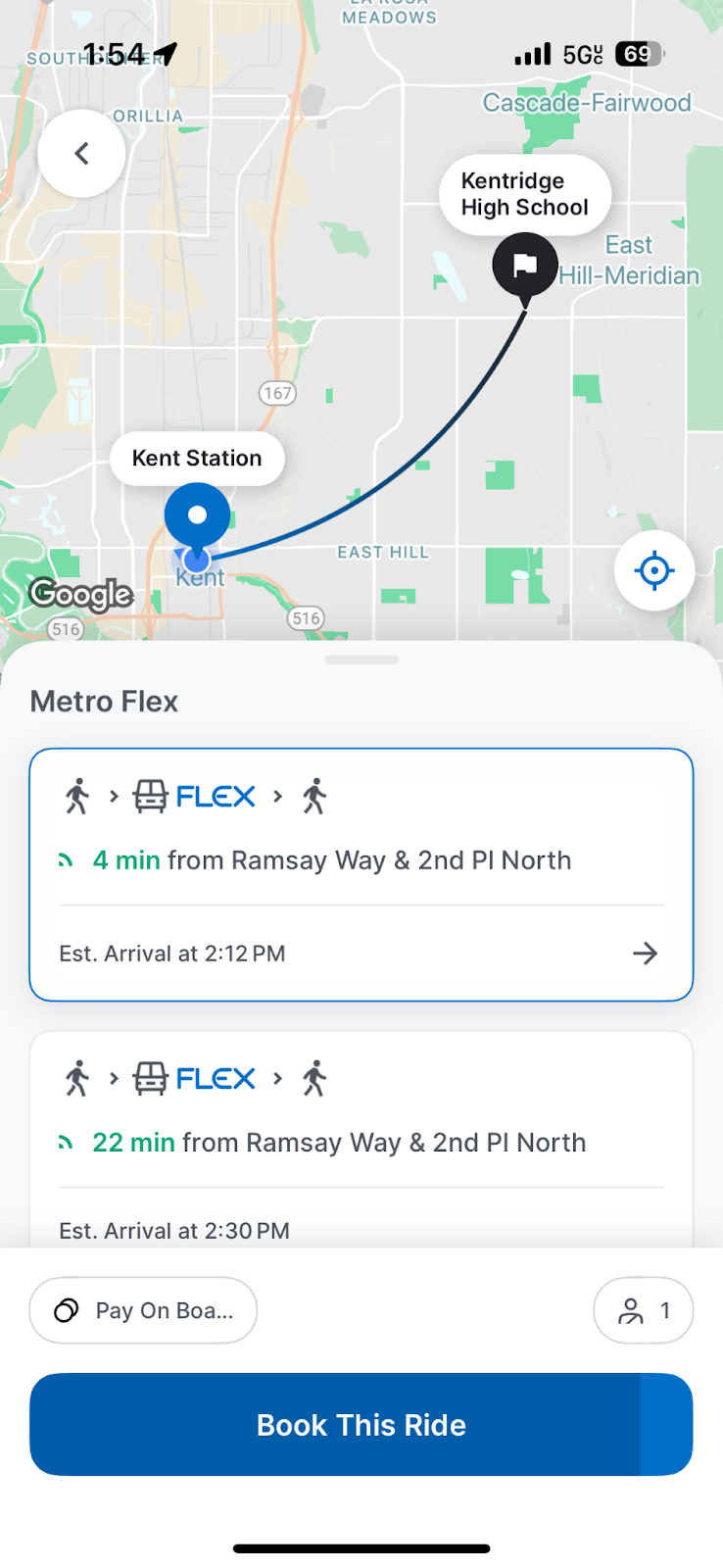The image appears to be a screenshot from an iPhone at 1:54 PM, with location services enabled and full 5G UC cellular signal. The battery level is at 69%. There is a back button present, suggesting navigation within an app. The app is a rideshare service, which is currently showing a route from Kent Station to Kentridge High School. Other nearby locations are highlighted, including Cascade Fairwood and East Hill Meridian.

Two ride options are displayed in detail. The first option, Metroflex, is 4 minutes away from Ramsey Way and Second Place North, with an estimated arrival time of 2:12 PM. The second option is 22 minutes away from the same starting point, with an estimated arrival at 2:30 PM. Both options indicate that they are for one person and offer an on-board payment method. At the bottom of the screen, there is a prominent blue button with white text that reads "Book this ride."